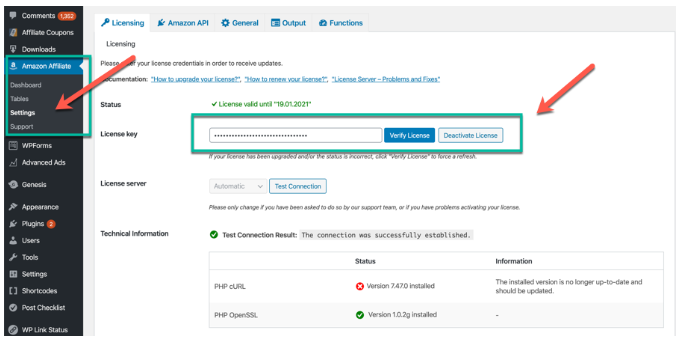This image displays a cropped screenshot of an admin panel and an application interface. On the left side, there is a black vertical banner showing a list of menu items in a column format, including "Comments," "Affiliate," "Coupons," and "Downloads." The "Amazon Affiliate" section is highlighted with a green box, indicating it is selected. Underneath the "Amazon Affiliate" title, additional options such as "Dashboard," "Terms," and "Settings" are listed, with "Settings" highlighted in white.

Adjacent to the "Settings" option, a red arrow is edited into the image to draw attention to it. On the right side, the page displays the "Settings for Licensing," with the header clearly stating "Licensing." The central area of the image prominently features a large green box overlaying the "Verify License" and "Deactivate License" buttons, with another red arrow pointing towards these options, emphasizing their importance.

Overall, the various elements—including highlighted sections, inserted arrows, and distinct color boxes—clarify the navigational flow and focal points within the admin panel.